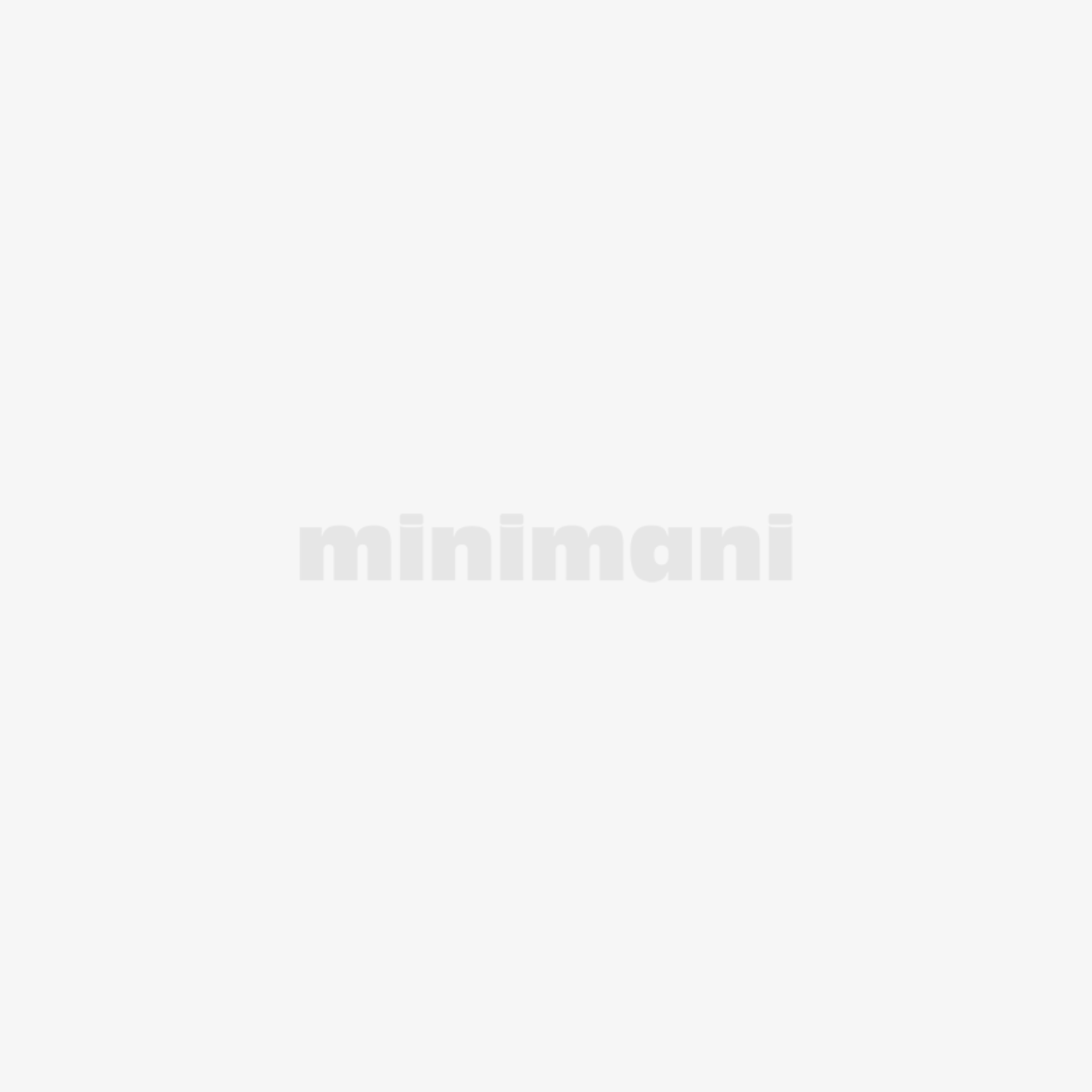This image features a stock photo of a red cardboard box positioned diagonally against a white background, typical of supermarket website displays. The box prominently features the brand name "Calvo" in large white font at the top, set against a blue label. Beneath the brand name, there is text in a foreign language (possibly listing ingredients or product description), followed by the English phrase "Tuna Steak in Tomato Sauce" underlined in white. The lower left corner features a pull-tab icon with the text "Easy Open." An image on the lower right portrays a round tuna steak, pale pink in color, resembling a hockey puck. Behind it, two ripe red tomatoes with green stems are visible, adding to the visual appeal. A small “serving suggestion” note is included at the bottom right corner.